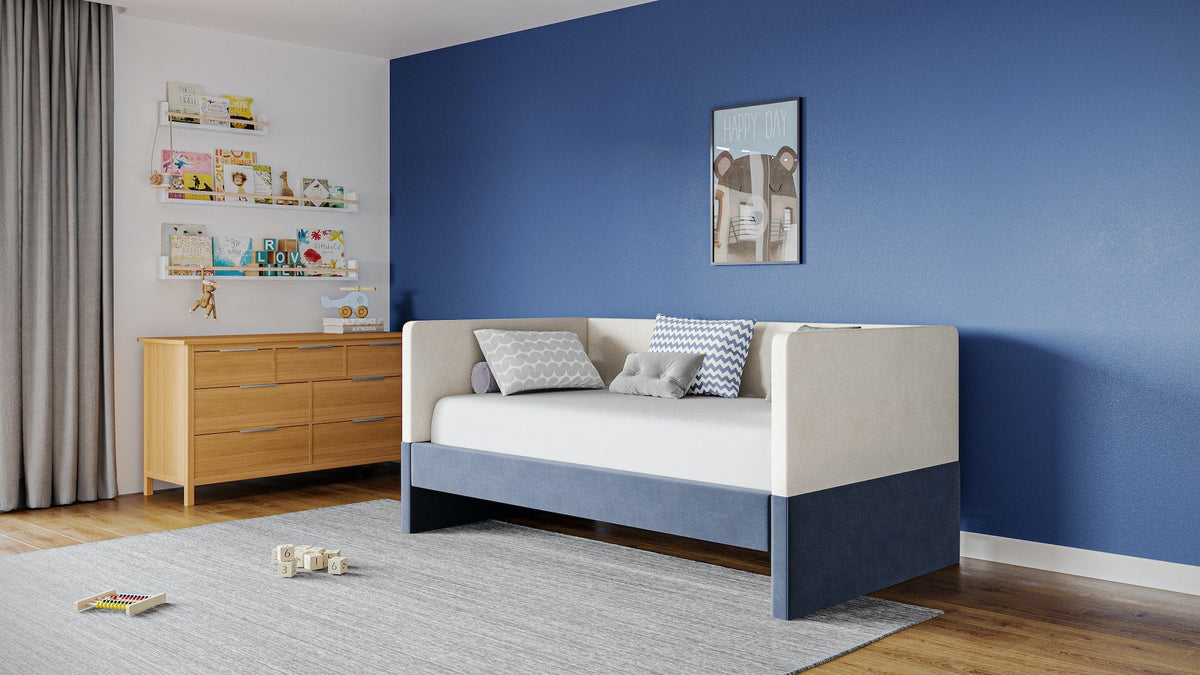The image depicts what appears to be a children's waiting room or a family-oriented room in a house. The room features a dark blue wall in the background with a white wall on the left. Central to the image is a daybed or sofa adorned with a white upper section and a dark blue lower section, complemented by four pillows—two large, one smaller, and one round. Above the sofa hangs a picture or illustration, potentially of a bear. To the left of the sofa stands a wooden sideboard unit with three shelves above it, populated by what seems to be children's books, including one partially reading "LOV." The hardwood floor hosts a large grey rug with a striped texture. Scattered on the floor are children's toys, including number blocks and an object resembling an abacus. Adjacent to the sideboard on the left, a grey curtain suggests the presence of a window behind it. The room also contains magazine racks filled with assorted magazines and toy items like a helicopter and a monkey, hinting at its family-friendly atmosphere.